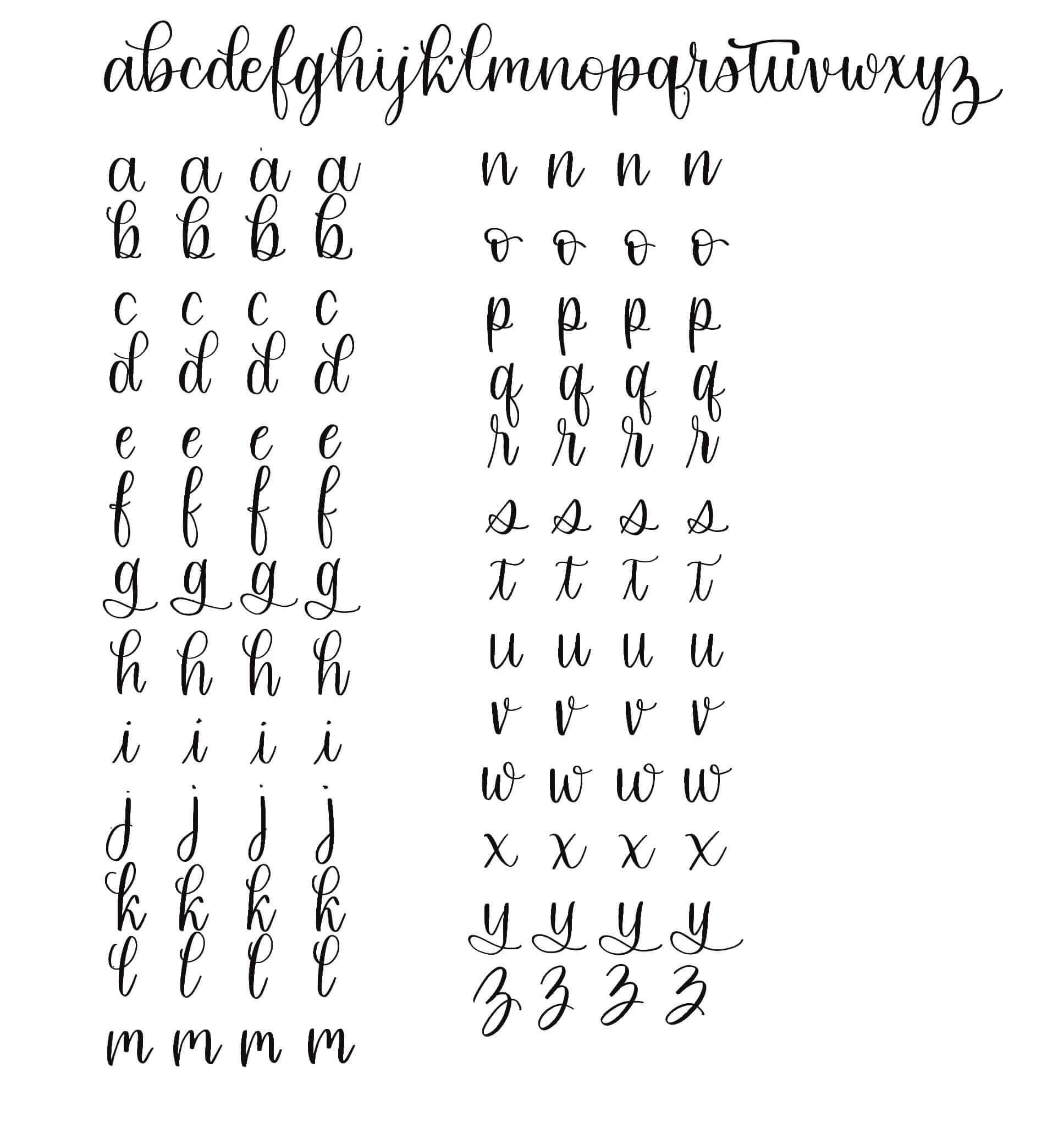This image is a detailed chart showcasing calligraphy practice, with black calligraphy handwriting on a white background. At the very top, the entire alphabet from A to Z is presented in cursive, with all the letters elegantly connected to form a continuous line. Below this, the chart is divided into two main sections for further practice. The left column features the letters A through M, each written four times, while the right column contains the letters N through Z, also written four times. Each letter in these columns stands alone, providing multiple examples of how to form each character individually. This arrangement serves as a comprehensive guide for learning and practicing calligraphy.